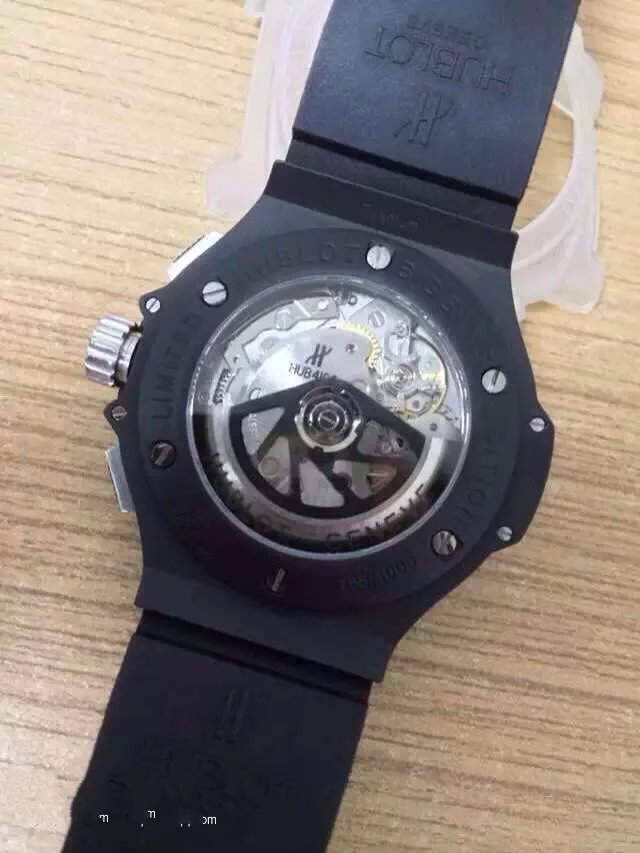This photograph depicts a sophisticated black watch with an intricate design, prominently featuring its inner clockwork mechanisms. The black watch band, likely made of a material other than leather, secures the watch to your wrist. The watch is displayed on a light brown wooden table, with visible wood grain adding texture to the background.

The central focus of the watch is its transparent face, showcasing the inner cogs and machinery, which combine silver and black elements. Surrounding the watch face are small silver screws and a silver dial knob on the side, possibly used for adjusting the time. There is faint text that appears partially visible, with the letters "H-U-B-L-O-T," suggesting the brand is Hublot.

Additionally, a clear, plastic-looking object is positioned at the top of the wristband, behind the watch. The detailed craftsmanship of the watch’s back side is also evident through the photograph, revealing the screws and machinery that secure it together. The image is solely focused on the watch, the band, the table, and the distinctive clear material, presenting a stark, minimalist composition.